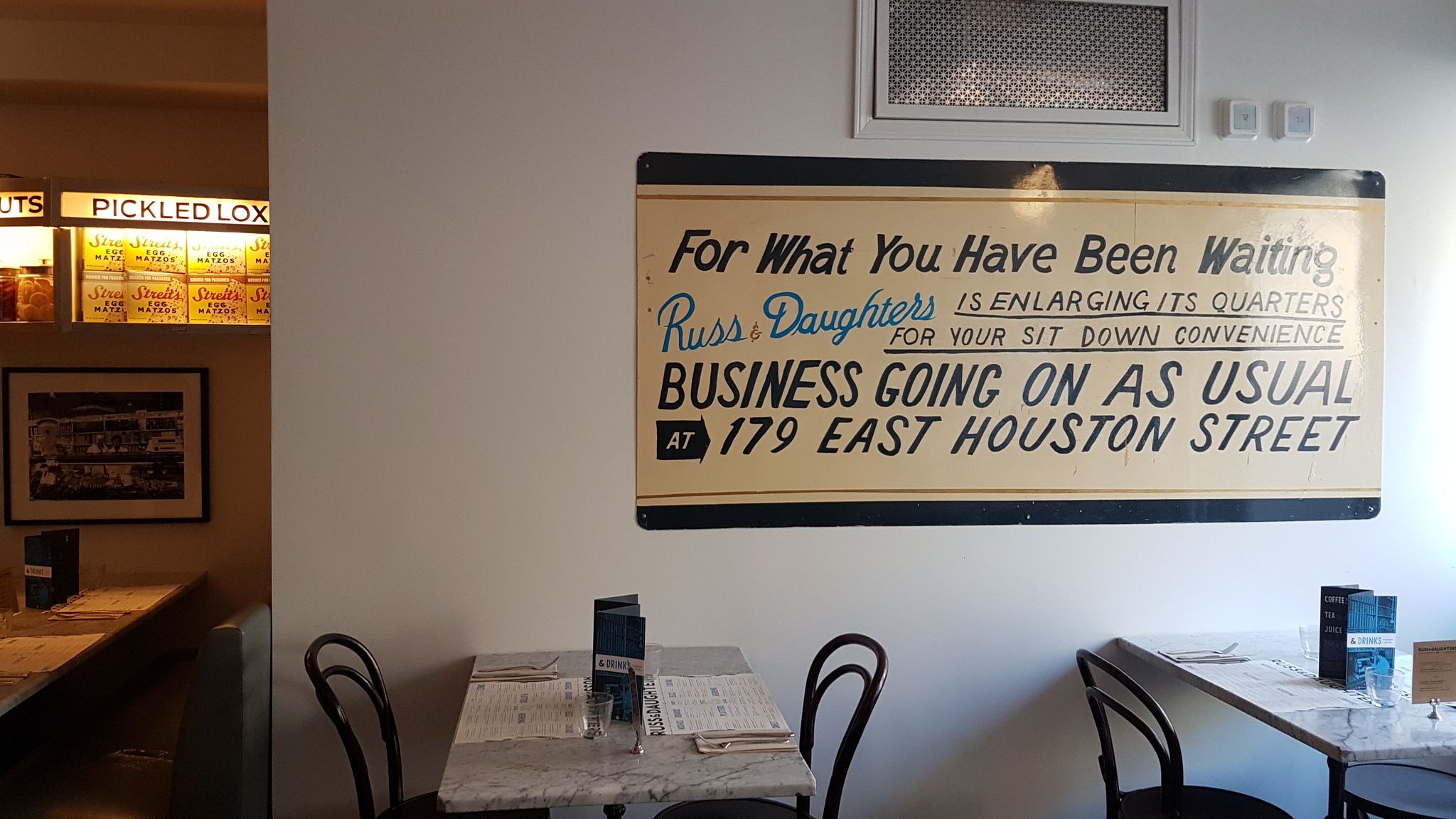In the image of the restaurant interior, two prominent white and black marble tables are seen, each accompanied by old, black bentwood chairs. The tables, positioned in the bottom-left and bottom-right of the image, have napkins with forks placed on them. There are menus and empty glasses visible, suggesting readiness for diners. Behind the tables, a white wall features a large, retro-styled rectangular poster. The poster, with a white background and dark letters, reads, "For what you have been waiting." In blue letters, it continues, "Rush Daughters is enlarging its quarters for your sit-down convenience. Business going on as usual at 179 East Houston Street." The sign also incorporates a blue arrow motif. To the left of the image are more counters and a photograph mounted on another wall. In the background, a lit sign that reads "Pickle Box" with backlighting highlights a list of other menu items. The overall ambiance is filled with retro elements and suggests a nostalgic theme, underscored by the vintage-styled signs and décor.